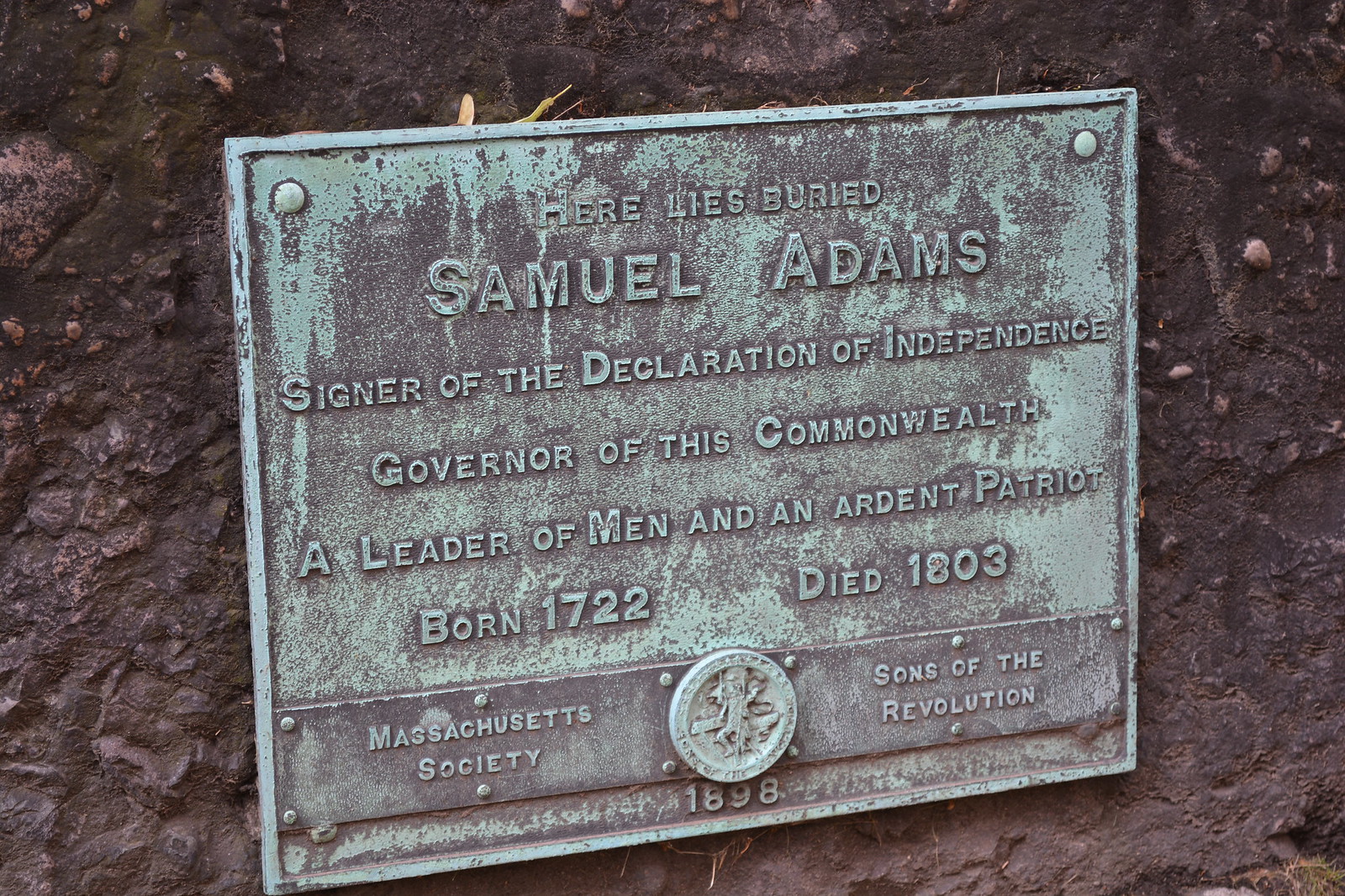This image features a detailed view of a historical gravesite marked by a naturally worn, stone outdoor wall obscured by dirt and twigs. At the center of the image is a metal plaque set against the stone. The plaque prominently reads, "Here lies buried Samuel Adams," followed by a series of inscriptions praising his accomplishments: "Signer of the Declaration of Independence," "Governor of this Commonwealth," "A leader of men and an ardent patriot." In smaller text, it states, "Born 1722, died 1803," and on the bottom left corner, "Massachusetts Society." On the right corner, it says, "Sons of Revolution," with the year "1898" inscribed at the very bottom, likely indicating the date of the plaque's dedication. Above this text, there is an emblem in the form of a circular icon. The scene is devoid of any other objects, emphasizing the solemnity of the gravesite. The colors in the image comprise earthy tones such as brown, yellow, green, tan, and gray, blending the natural elements with the aged stone and metal.